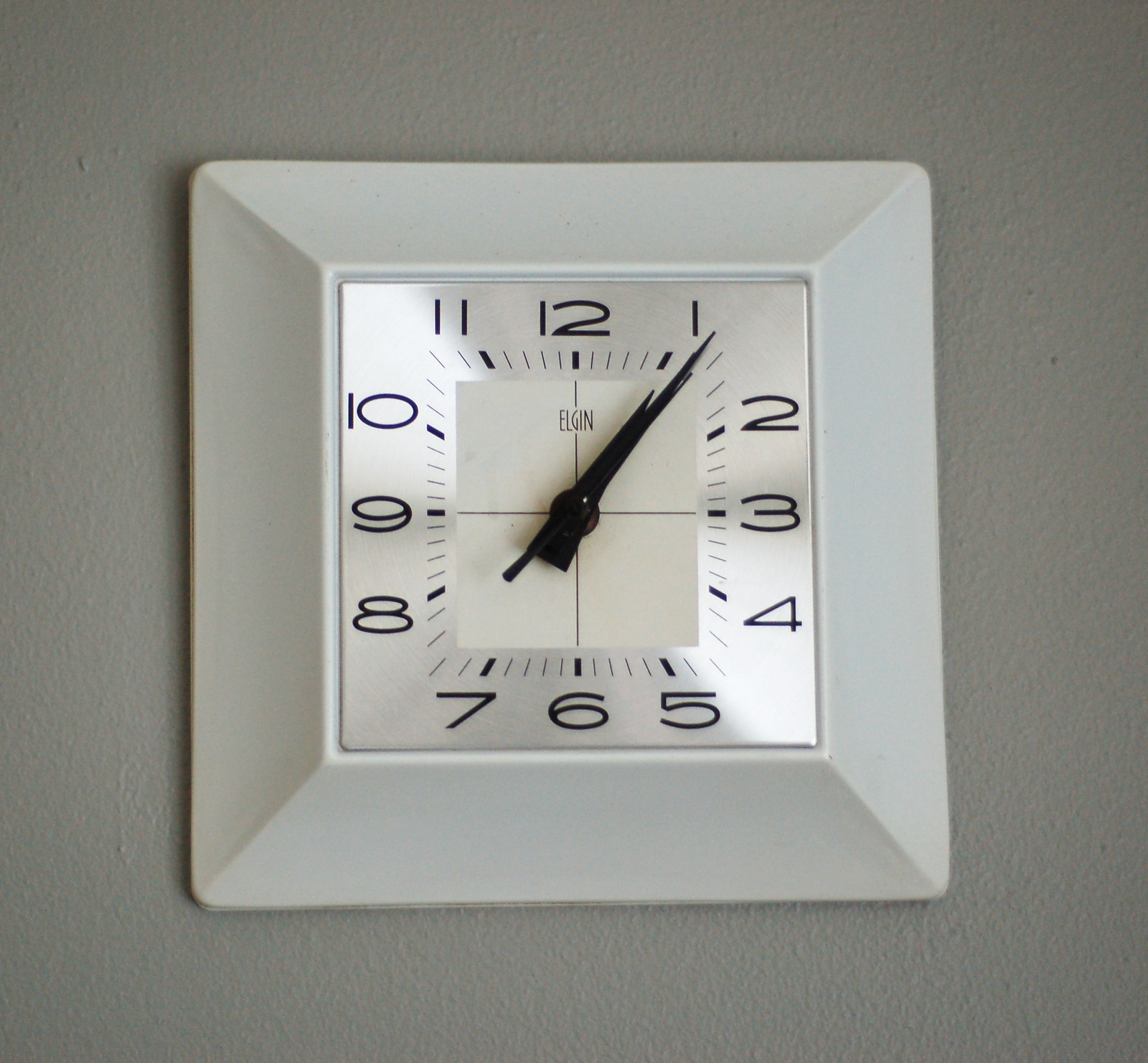This is a color photograph of a square-shaped white clock hanging on a gray wall. The clock, centrally framed and occupying most of the image, features a shiny, metal-like white face with an inner square divided into four smaller squares. The clock is enclosed in a slightly elevated white ceramic frame, resembling an upside-down square dinner plate. The black hands of the clock, including the hour, minute, and second hands, are pointed just past the number one, indicating the time as 1:06. The clock displays large, simple black numbers arranged in a unique pattern around its perimeter: 11, 12, and 1 appear at the top from left to right; 2, 3, and 4 are on the right side from top to bottom; 7, 6, and 5 are at the bottom from left to right; and 10, 9, and 8 are on the left from top to bottom. The brand name "Elgin" is printed just beneath the 12, and there are small marks indicating the minute increments.